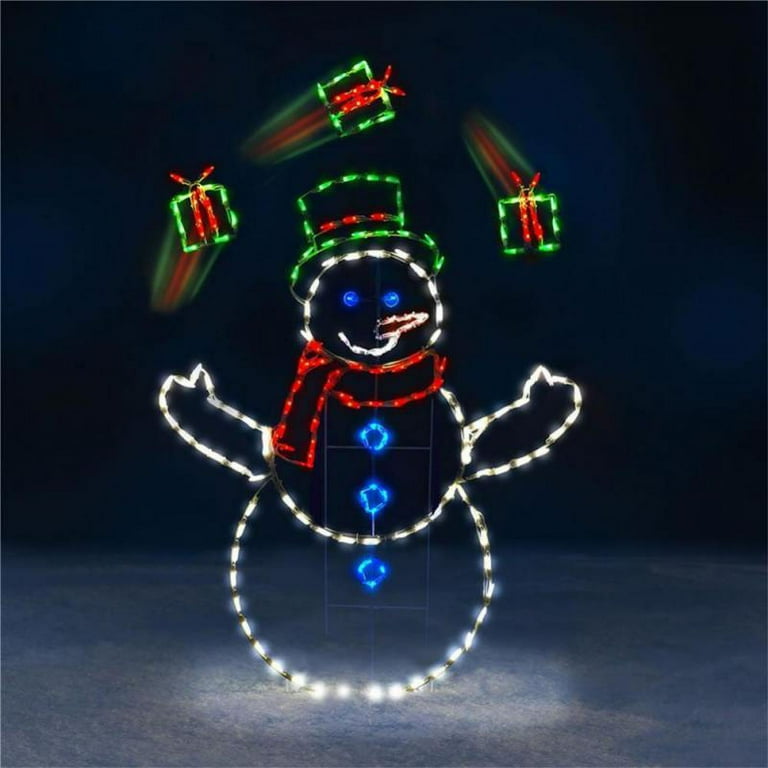The image is a detailed photograph of a snowman holiday light display set against a dark night sky. The snowman is outlined in white LED lights, with three distinct sections forming its body and arms. His head, complete with a blue-eyed, white-lit smile and a brown-accented, white-lit carrot nose, is topped by a green hat with a red band. A red-lit scarf drapes around his neck, hanging to the left, adding a festive touch.

The snowman is seen juggling three Christmas presents, each outlined in green lights with red vertical stripes in the middle and red bows on top. These presents have green and red light streaks behind them, creating a dynamic effect that suggests motion. The presents are positioned above the snowman's head and arms, with one above the head and one above each hand. 

The snowman stands on a white, snow-covered surface, adding to the wintry scene. The entire display is set against a dark blue background, evoking the feeling of nighttime during the holiday season.